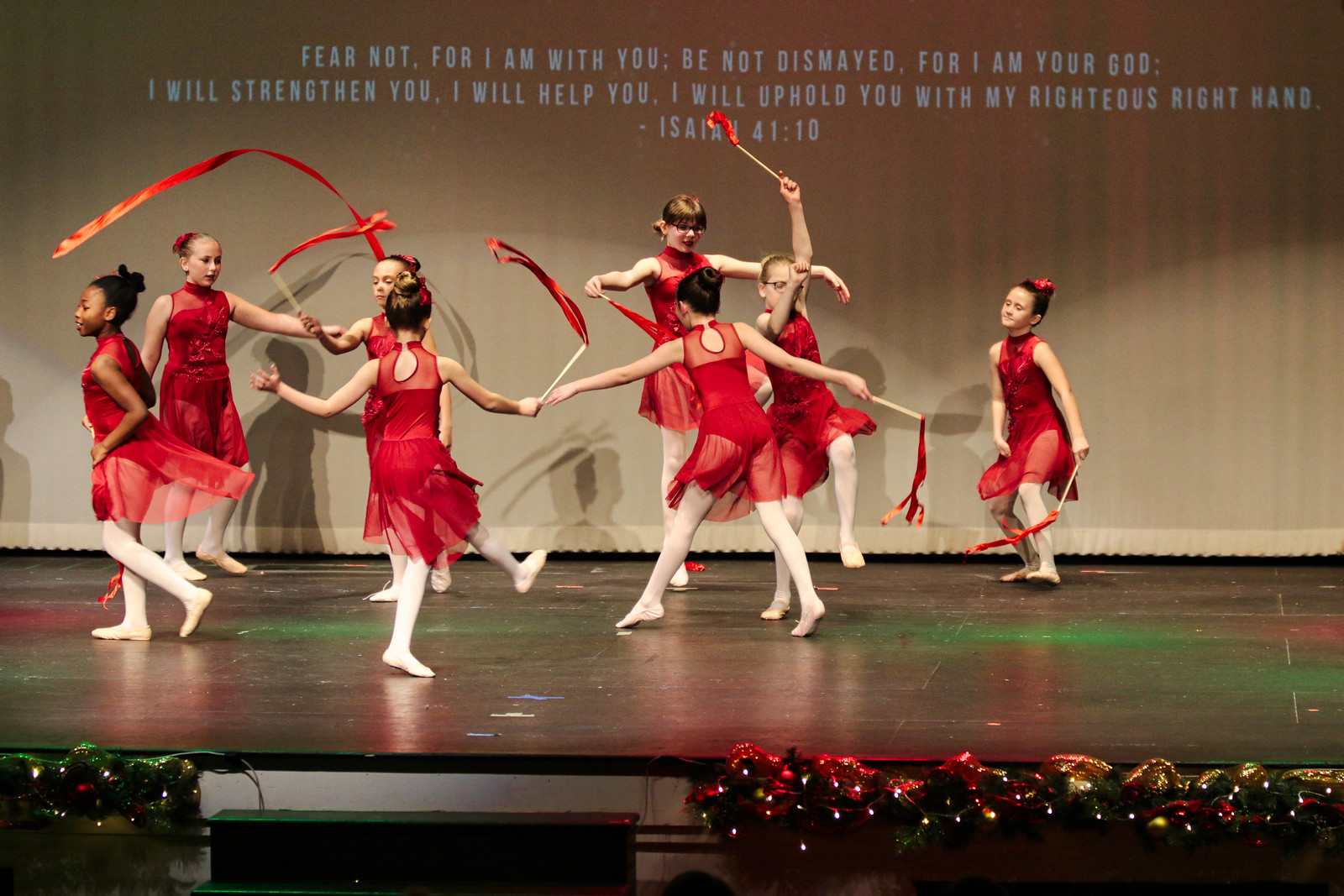This indoor photograph captures a group of young, female dancers, likely aged 11-12, performing on a wooden stage. Dressed in coordinated red outfits, each dancer wears a sheer red skirt and a matching leotard adorned in a style reminiscent of Chinese dresses, complemented by white stockings. The girls are seen twirling red ribbons in a graceful ballet performance, set against a backdrop where a Bible quote is projected on the wall behind them. The text reads, "Fear not, for I am with you. Be not dismayed, for I am your God. I will strengthen you. I will help you. I will uphold you with my righteous right hand. Isaiah 41:10." The festive atmosphere is enhanced by Christmas light decorations adorning the front edge of the stage, except for an area at the center left where steps lead down from the stage. There are approximately eight or nine dancers in total, all contributing to this vibrant and heartfelt performance.